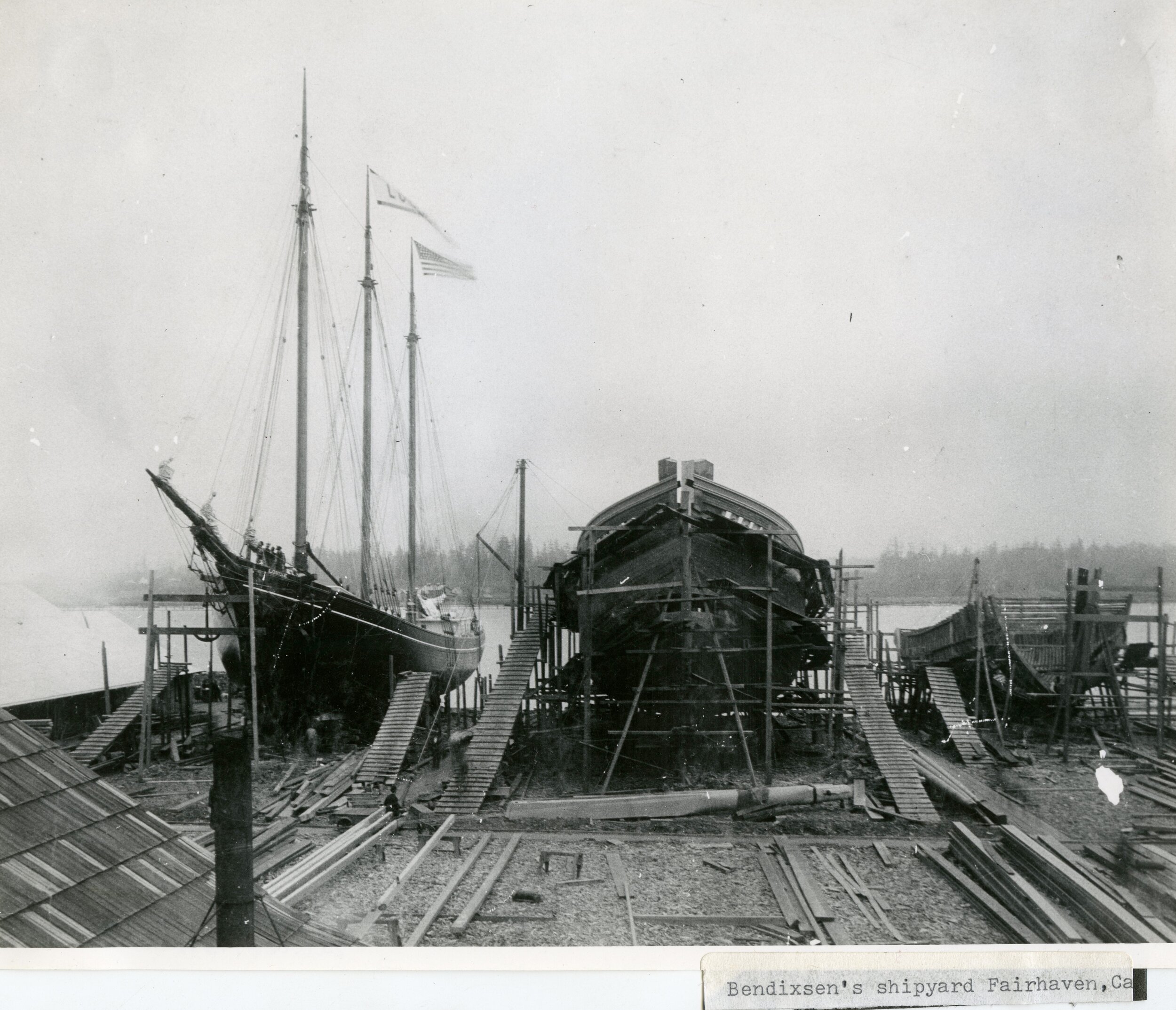A vintage black and white photograph capturing the historic Ben Dixon's Shipyard in Fairhaven, California. The image portrays three partially constructed ships prominently positioned on a dock that is also under construction. Each ship is encased in a meticulous wooden skeletal framework, indicative of their ongoing assembly. Wooden planks, resembling scaffold-like ramps, extend up to the ships, facilitating workers' access to various parts of the vessels. The scene, frozen in time, reflects the industrious spirit of early 20th-century shipbuilding.